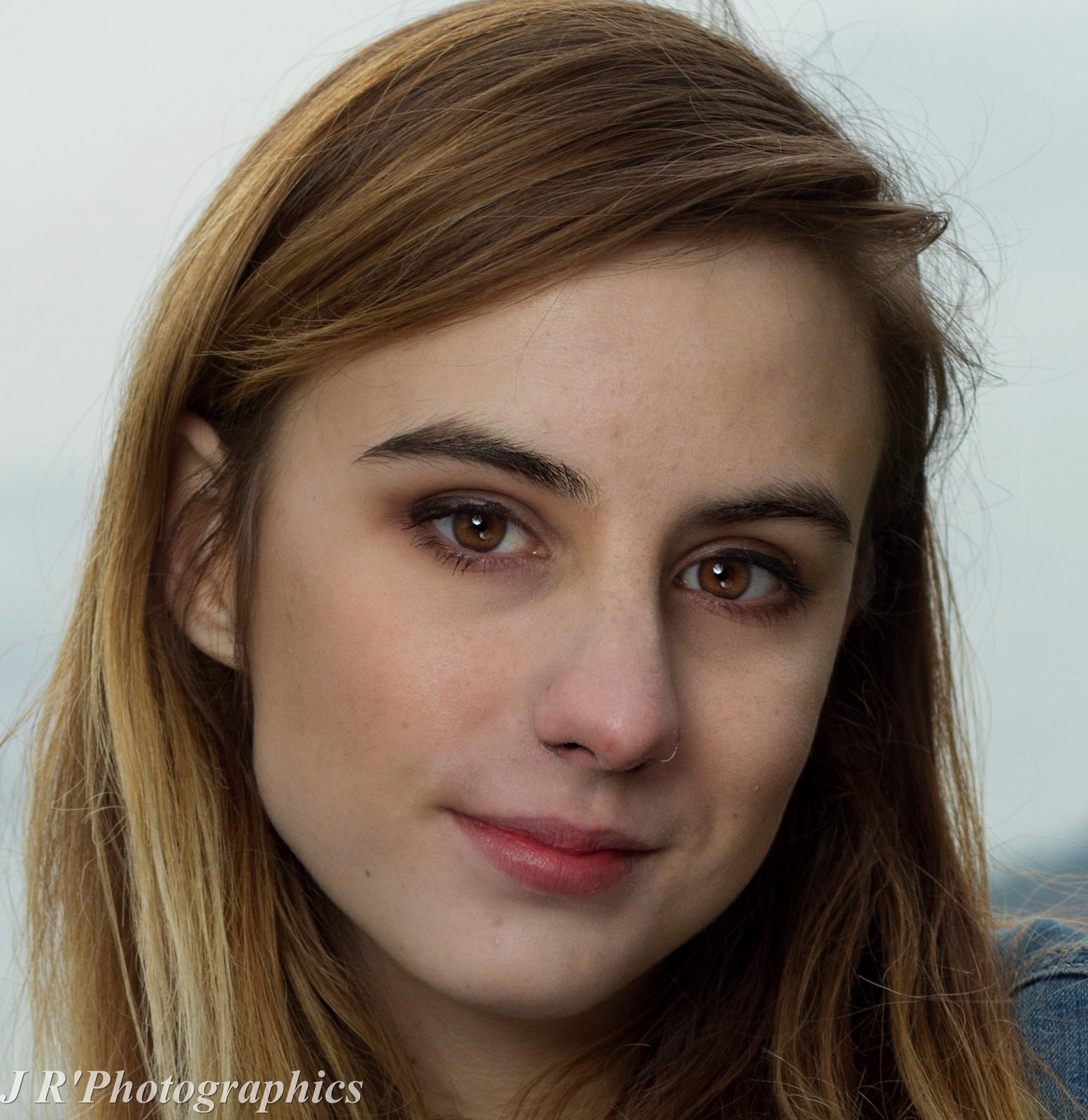This is a detailed headshot of a young woman, likely in her early to mid-20s, with natural minimal makeup. Her brown hair, featuring numerous blondish highlights and subtle reddish tones, extends to her shoulders, partially covering her ears. She has brown eyes and darker brown eyebrows, and her lips are pursed as she gazes directly into the camera. She is wearing a blue denim jacket or shirt, and the background appears to be a soft, light gray or white, giving a neutral backdrop to her features. A watermark reading "J.R. Photographics" is visible in the lower left corner, suggesting this could be a professionally taken portrait.